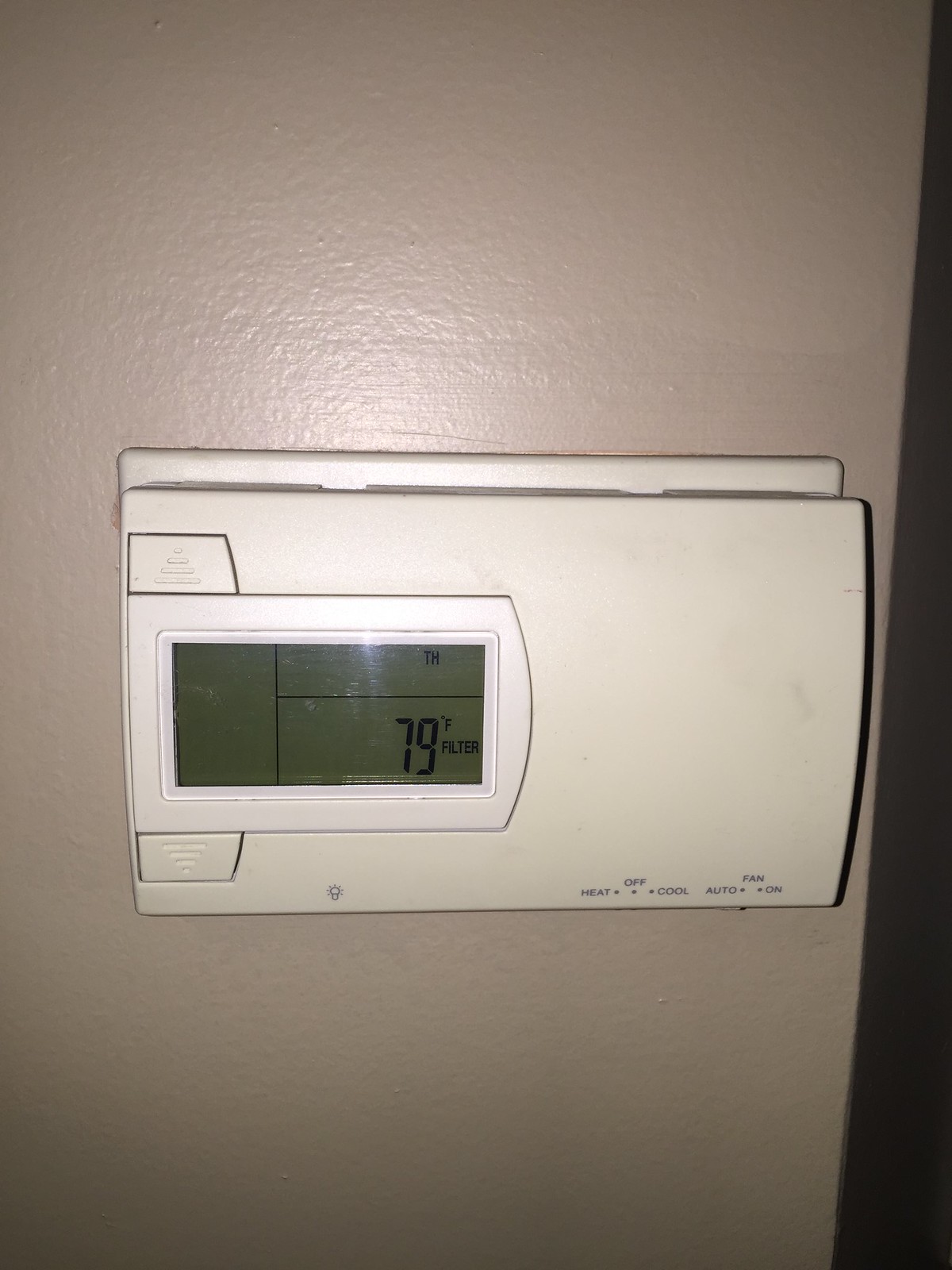The image features a mounted thermostat situated on a beige-colored wall. The wall paint, flat and non-reflective, is subtly highlighted by a camera flash. The thermostat, positioned sideways, stands as the focal point, displaying a current temperature reading of 79°F.

This rectangular white device has a slightly smudged surface from fingerprints, and it is detailed with a horizontal LED screen. Several zones of this screen convey crucial information: the upper left segment indicates 'HEAT,' while directly below '79°F' and 'FILTER' are prominently shown. The LED display is bordered by a white frame, with distinct divisions made by black lines to compartmentalize the information.

On the left side of the thermostat, a button, slightly wider at the bottom and featuring four indents for grip, allows for temperature adjustments. Below the screen, a similar button is present, maintaining the design continuity with identical grip indents.

At the very bottom of the thermostat, a control switch offers different ventilation options. The symbols in black include a star icon denoting light functionality and a fan symbol with 'AUTO' and 'ON' settings. Adjacent to these is a switch for temperature mode adjustments, labeled with 'HEAT' on the left, 'OFF' in the center, and 'COOL' on the right.

Overall, the detailed design and functional elements of the thermostat are clearly visible, creating a comprehensive visual guide to its various buttons and displays.